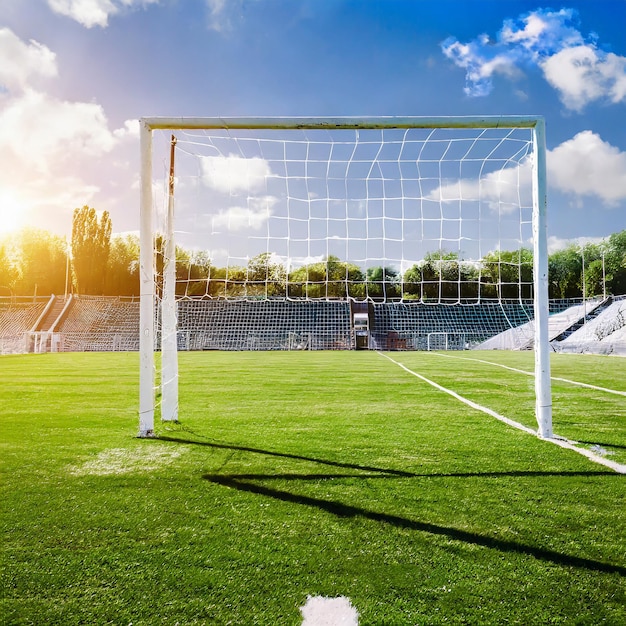This photograph captures a sunny, early dusk scene at a sports stadium, possibly AI-generated, depicting a meticulously maintained soccer field. The bright blue sky is adorned with puffy white clouds, and the sun, appearing on the left, casts a golden hue that hints at the start of a sunset. A row of trees of varying heights and thickness lines the horizon, just beyond the spectator stands. The stands, likely seating for several hundred, stand empty, framed by a fence running parallel in front of them.

In the foreground, a soccer goal post dominates the image. The net is white and attached at the top to white poles, but intriguingly, it seems to sag or stop partway down, casting a distinct shadow on the emerald green grass below. Adding to the unusual perspective, the goal post appears shifted, possibly due to photographic manipulation. Crisp white boundary lines are visible on the right side of the field, enhancing the organized and well-kept appearance of the venue. The overall scene exudes a calm yet vibrant atmosphere, with the lush green grass, the structured seating, and the vivid sky creating a picturesque sports setting.